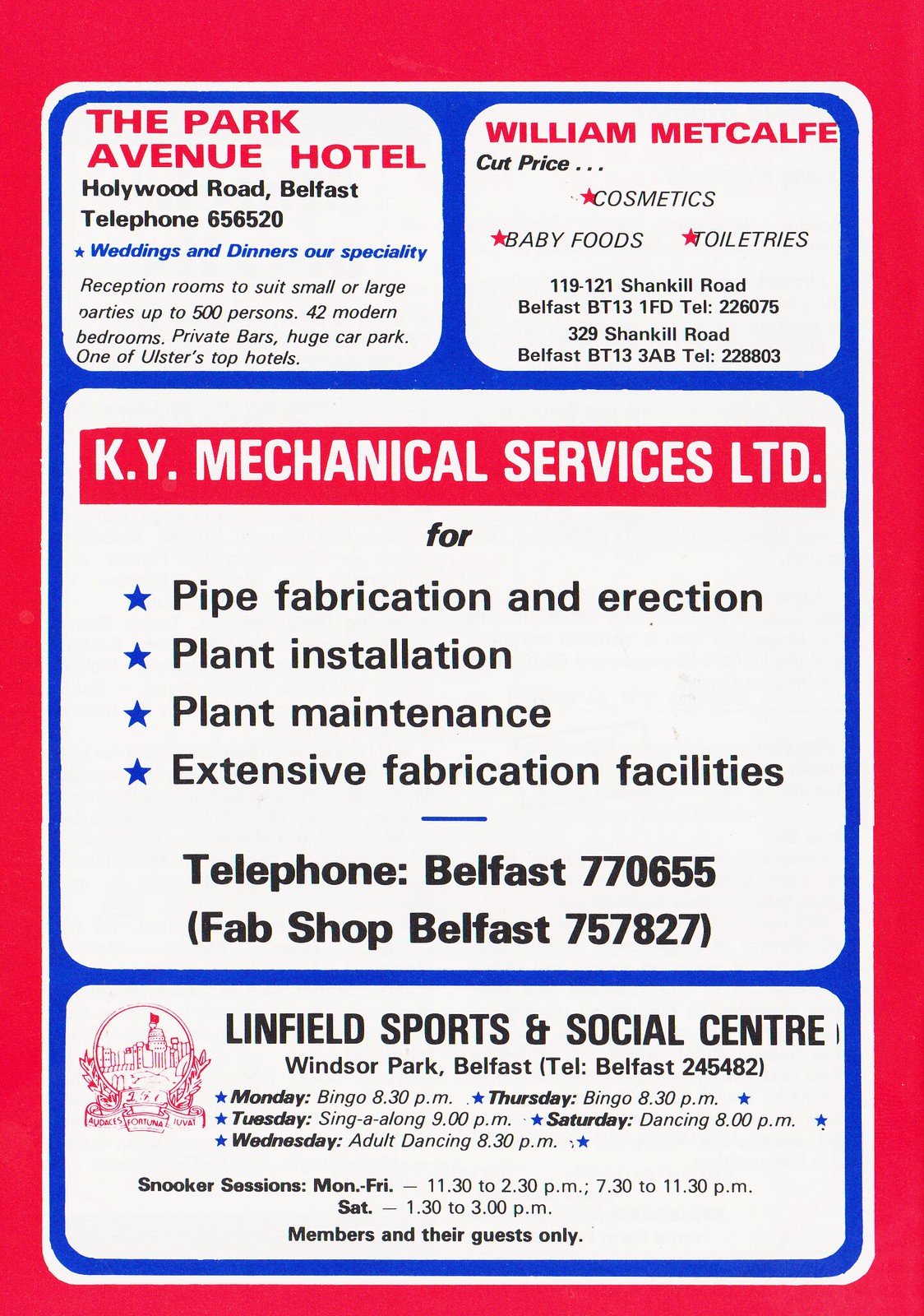The image depicts a red-bordered page containing four distinct advertisements, each encased in a blue-bordered box. The top-left ad promotes the Park Avenue Hotel, featuring a red header "The Park Avenue Hotel," followed by the address "Hollywood Road, Belfast," and the telephone number "656520." It also mentions "Weddings and Dinners Our Specialty" in blue.

The top-right ad is for William Metcalf, highlighted by a red title and keywords like "cut price," "cosmetics," "baby food," and "oil trees" accompanied by red stars. The contact details include addresses "119-121 Shank Hill Road, Belfast BT13 1FD" and "9 Shank Hill Road, Belfast BT13 3AB," with telephone numbers "2607 532" and "28803."

The central and largest ad on the page is for KY Mechanical Services LTD. It features white text on a red background and details their services: "Pipe Fabrication and Erection," "Plant Installation," "Plant Maintenance," and "Extensive Fabrication Facilities" alongside four blue stars. Their contact numbers are "Belfast 770685 (fab shop) Belfast 757827."

At the bottom is an ad for Linfield Sports and Social Center located in Windsor Park, Belfast. It lists open days, "Monday, Tuesday, Wednesday," and "Thursday, Saturday," with activities like snooker sessions, indicating "Monday through Friday," and "Saturday members and their guests only." The ad includes black text and a red design or logo.